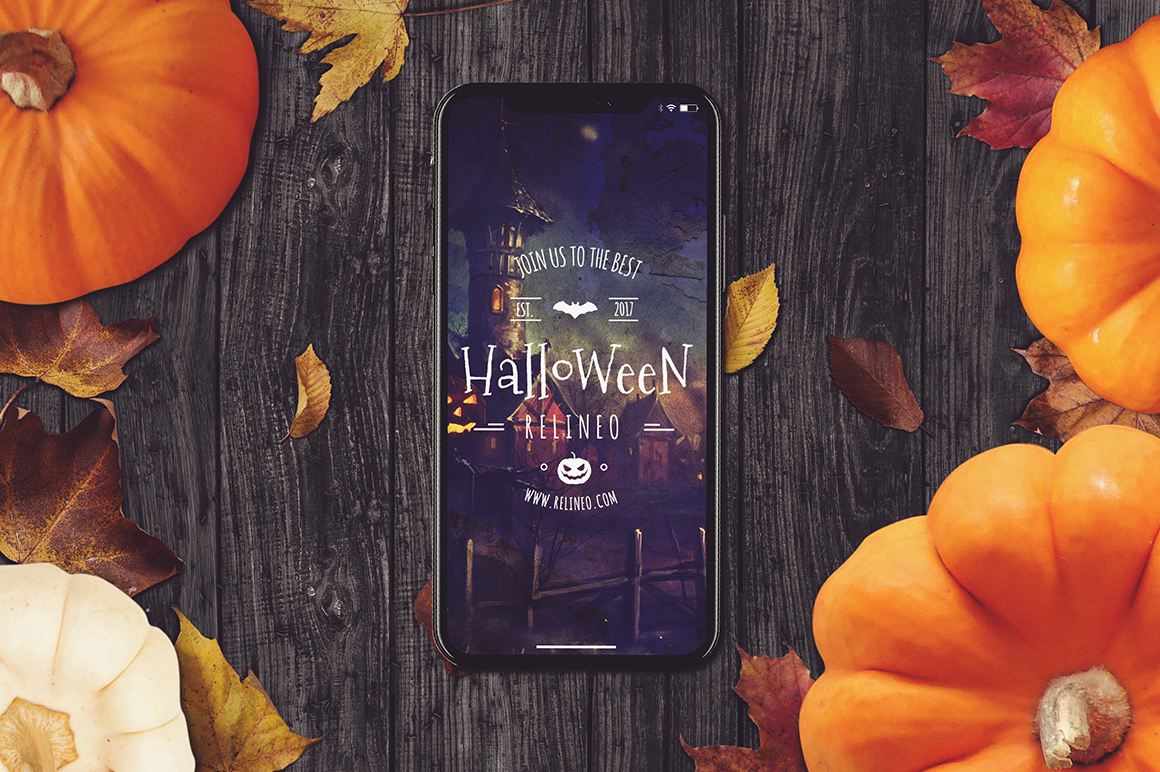The image depicts a cell phone positioned face-up on what seems to be a wooden surface, either a tabletop or a bench. The arrangement includes seasonal decorations: the four corners of the image showcase pumpkins or gourds. In the upper left, upper right, and lower right corners, the pumpkins are bright orange, while the lower left corner features a pumpkin or gourd in a creamy white color. Interspersed among these pumpkins are autumn leaves, scattered across the wooden surface, ranging in hues of orange and brown, some of which appear to be maple leaves.

On the screen of the cell phone is a dark, nighttime scene of a town, featuring a medieval tower to the left. Prominently displayed on the screen is a Halloween-themed graphic, including the illuminated face of a carved pumpkin, which is approximately the same size as one of the houses in the scene. The graphic text in the foreground reads, in white font: "Join Us to the Best Halloween Relineo," with an additional small pumpkin face icon beneath it. Below this, the URL "www.RELINEO.com" is presented in all caps.

Further details on the cell phone screen include text arranged in a circular pattern below "Join Us to the Best," enclosing a white bat icon. To the left of the bat icon are the letters "EST." (short for established), and to the right, the year "2017," both in white.